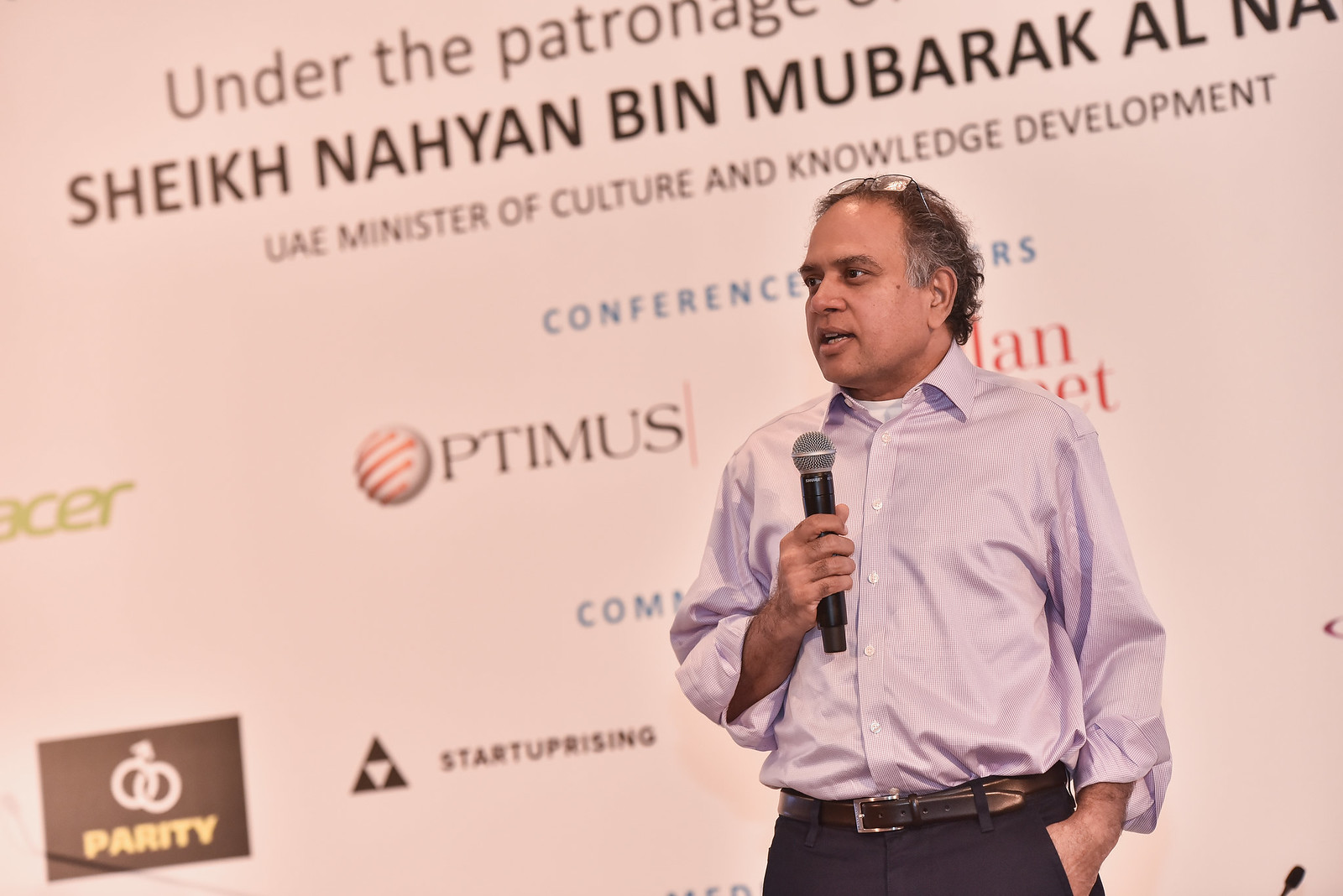The photograph depicts a man of Indian descent standing and speaking at what appears to be a convention, in front of a white backdrop adorned with several logos. The backdrop has a partially visible banner that reads, "Under the Patriot of Something. Sheikh Nayan Bin Mubarak Al," followed by "UAE Minister of Cultural and Knowledge Development," though the text is somewhat blurry. The man is dressed in a business casual manner, wearing a white and blue (or light purple) striped button-up shirt with a white undershirt beneath it. His shirt is tucked into dark blue business pants, secured with a black belt. He has rolled up his sleeves and is holding a microphone in his right hand. His glasses are perched on top of his head, nestled in his thin, dark hair with graying around the ears. The man is looking and speaking towards the left side of the image, and a secondary, smaller microphone is visible at the bottom right corner of the photo, likely mounted on a podium.